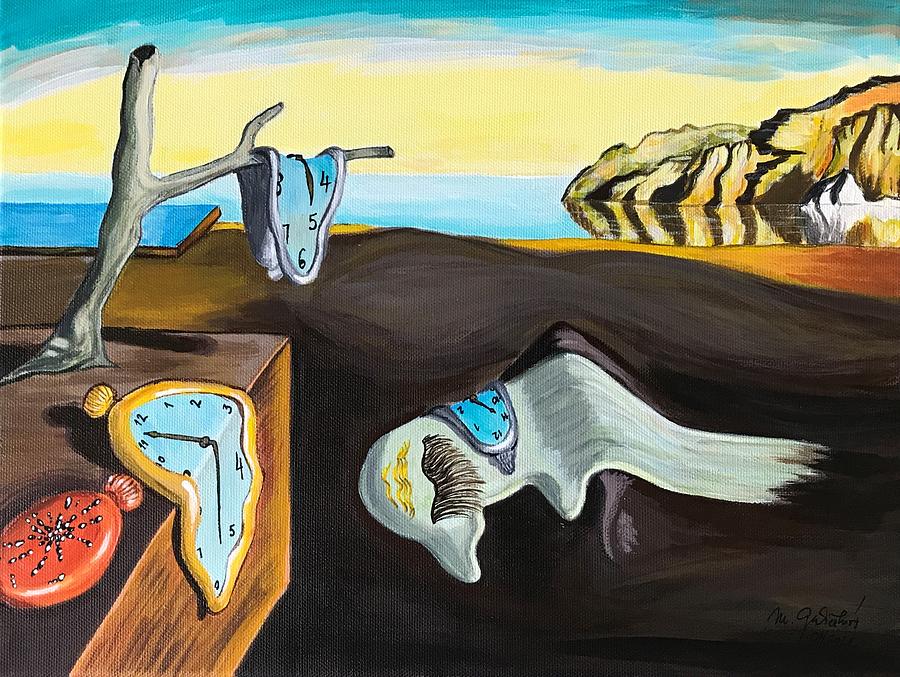This detailed depiction is a reinterpretation of Salvador Dalí's famous painting, "The Persistence of Memory,” serving as an environmental statement. The horizontal psychedelic illustration showcases a surreal landscape with a blue sky and yellow horizon, transitioning into blue water. To the right, a higher elevation in yellows, tans, gold, and orange emerges, which is thought to symbolize a once glacier-covered mountain now fully exposed, with a small remnant iceberg beside it, reflecting off the water.

In the foreground, surreal melting clocks dominate the scene. A gold clock with a blue interior drapes over a barren tree branch, while a silver clock, also blue inside, bends on the ground. Another silver clock grotesquely melts over what appears to be an illustrated dead bird with closed eyes and long lashes, lying on a desolate beach composed of dark browns and whites. 

At the lower left, a large box hosts another melting timepiece, set to 11:30, with an unopened orange clock beneath it. A bare tree trunk sprouts from the box, extending a limb with yet another melted watch. Additionally, a red oval container grows from the box's base.

Hidden throughout the painting are paint marks indicating it is an impression with only the bottom left part of "The Persistence of Memory" highlighted. The artist’s signature, "Mr. Gar Save Hers," found in the lower right corner, implies a call to action about the urgency of environmental preservation.